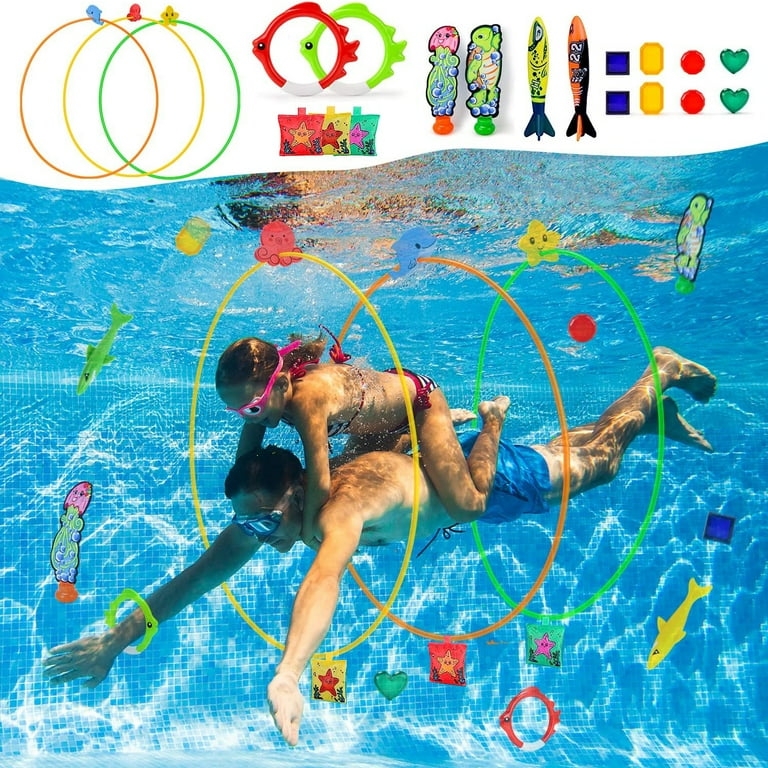In a vibrant underwater scene, a young girl clutches her father's shoulders as he swims through suspended hoops in a colorful pool. Both are equipped with goggles; she wears pink ones and a red striped bikini, while he sports larger goggles and blue swim trunks. The hoops they navigate are colored yellow, orange, and green, each supported by whimsical, smiling toys shaped like octopuses, dolphins, and stars. Above the immersive underwater activity, various pool toys are displayed, including hoops, rings, plastic fish, torpedoes, and gem-shaped objects, all available for purchase. The pool's yellow-tiled environment sparkles with light reflections, emphasizing the playful and vibrant nature of the scene. The abundance of bright colors—greens, oranges, and reds—enhances the visibility and appeal of the pool toys, creating a lively and engaging advertisement.